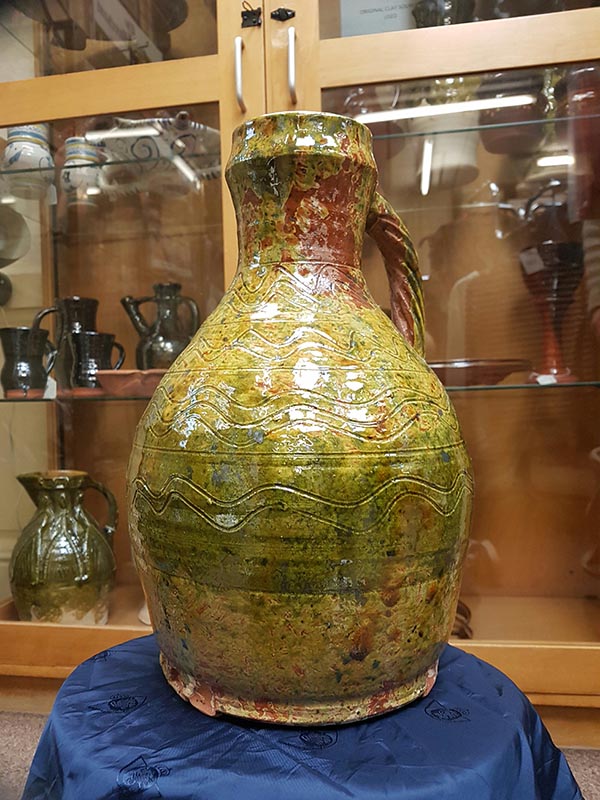This photograph showcases a lime green, yellow, and rust-colored ceramic vase with a distinct handle that curves upward, situated on a circular table covered with a blue, navy silk cloth. The vase, with its shiny enamel coating, features a large round bottom that narrows into a medium-sized opening, adorned with squiggly lines across its surface. Behind it stands a brown cabinet with glass doors and shelves, displaying an array of other vases and glassware in various shapes and sizes, including an army green vase with a spout. The cabinet's shelves hold an eclectic mix of pottery and glass items in hues like green, metallic silver, white, and red, indicating a store setting with numerous pieces of art on sale.